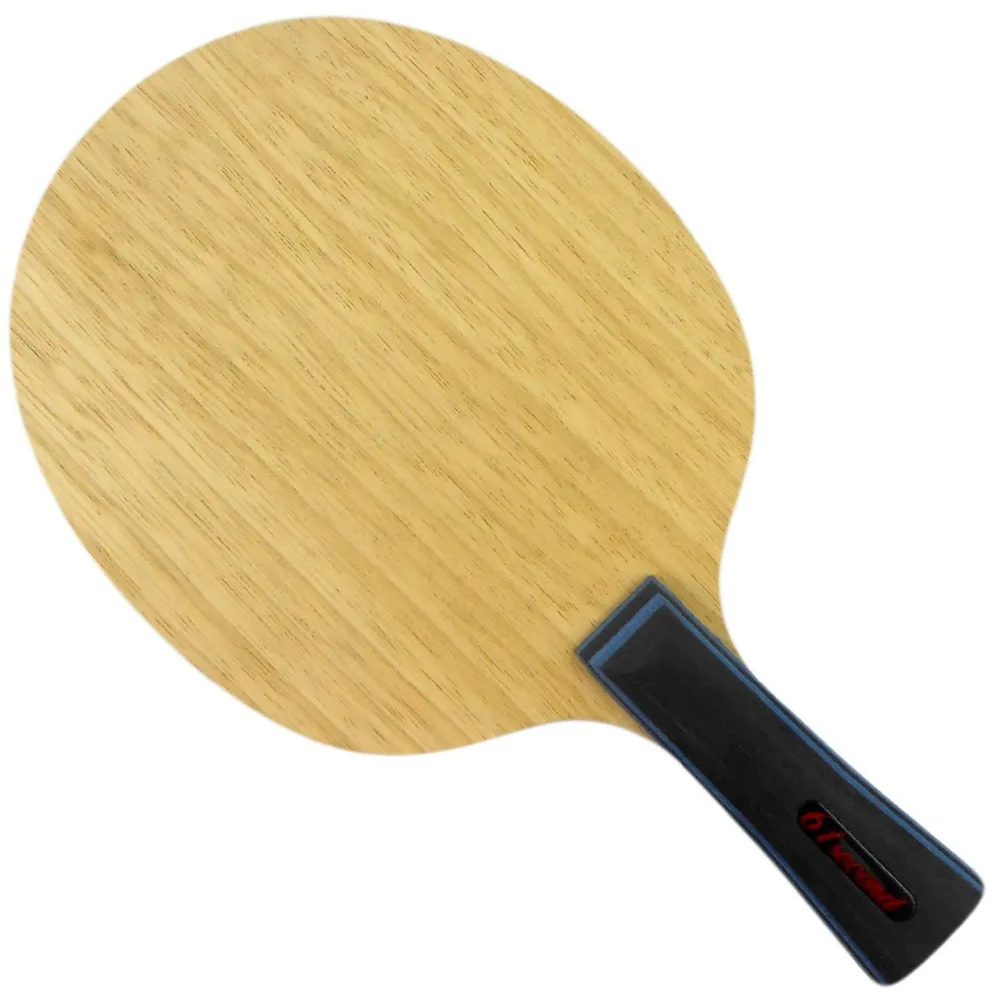This is a close-up image of a paddle, possibly used for paddleboarding, pickleball, or ping-pong. The paddle is made of a light-colored wood, likely bamboo or a light maple, exhibiting fine wood grain. The handle of the paddle is black with a light blue border around its top part, and it features some red text that is slightly blurry, making it hard to discern whether it forms a letter B or the number 6. The paddle itself is flat and has an oval or ovate shape. The background of the image is white, and the paddle is centered in the photo with no watermarks, trademarks, or other distinctive features in the setting.